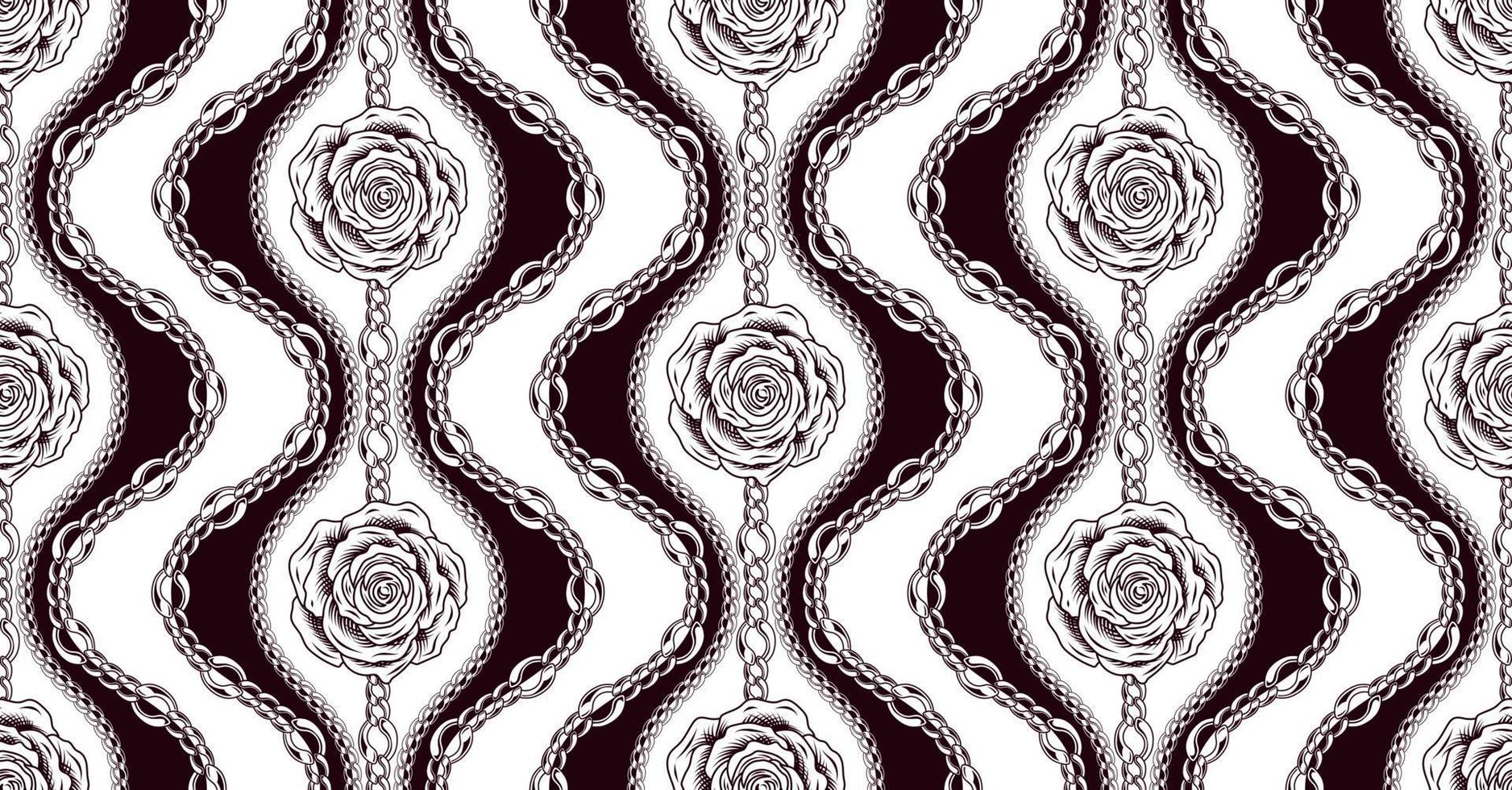The image is horizontally oriented and features an intricate, repetitive pattern that appears computer-generated, making it reminiscent of wallpaper or gift wrap. The design is predominantly black and white, almost resembling a photograph. Central to the pattern are roses, depicted in rows, either in sets of three or two, and displayed at an upright angle. Surrounding each rose is a silver and white chain that adds a dynamic, swirling effect to the visual. These chains form looped, circular bands around the roses, which in turn are set against a background with alternating dark strips. These strips wind down in a wavy, ribbon-like manner, interspersed with bulbous cylinders that create a beaded appearance, leading from top to bottom. The absence of text keeps the focus solely on this visually busy yet elegant pattern, which could be the artistic work of a tattoo artist or a detailed digital creation.